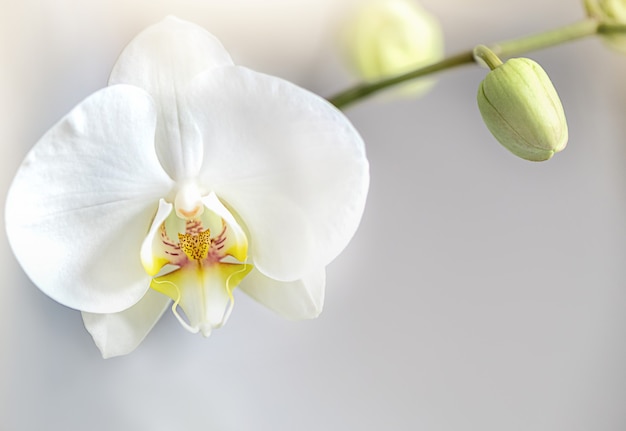This close-up outdoor photograph captures a striking white orchid in full bloom, positioned on the left side of the image. The orchid features five prominent petals: two extending horizontally, and three vertically arranged with one petal extending straight upward and two more diagonally positioned at the bottom. The petals are reminiscent of insect wings, enhancing the flower's intricate beauty. The flower's center displays a captivating gradient of white, yellow, and purple, with a distinct structure that resembles an open mouth with a protruding tongue. To the right of the flower, the green stem extends horizontally from right to left, supporting two unopened green buds poised to bloom. The background is a soft, blurred mixture of white, gray, and blue hues, devoid of any text or people, bringing full attention to the orchid's detailed morphology and the anticipation of its future blossoms.